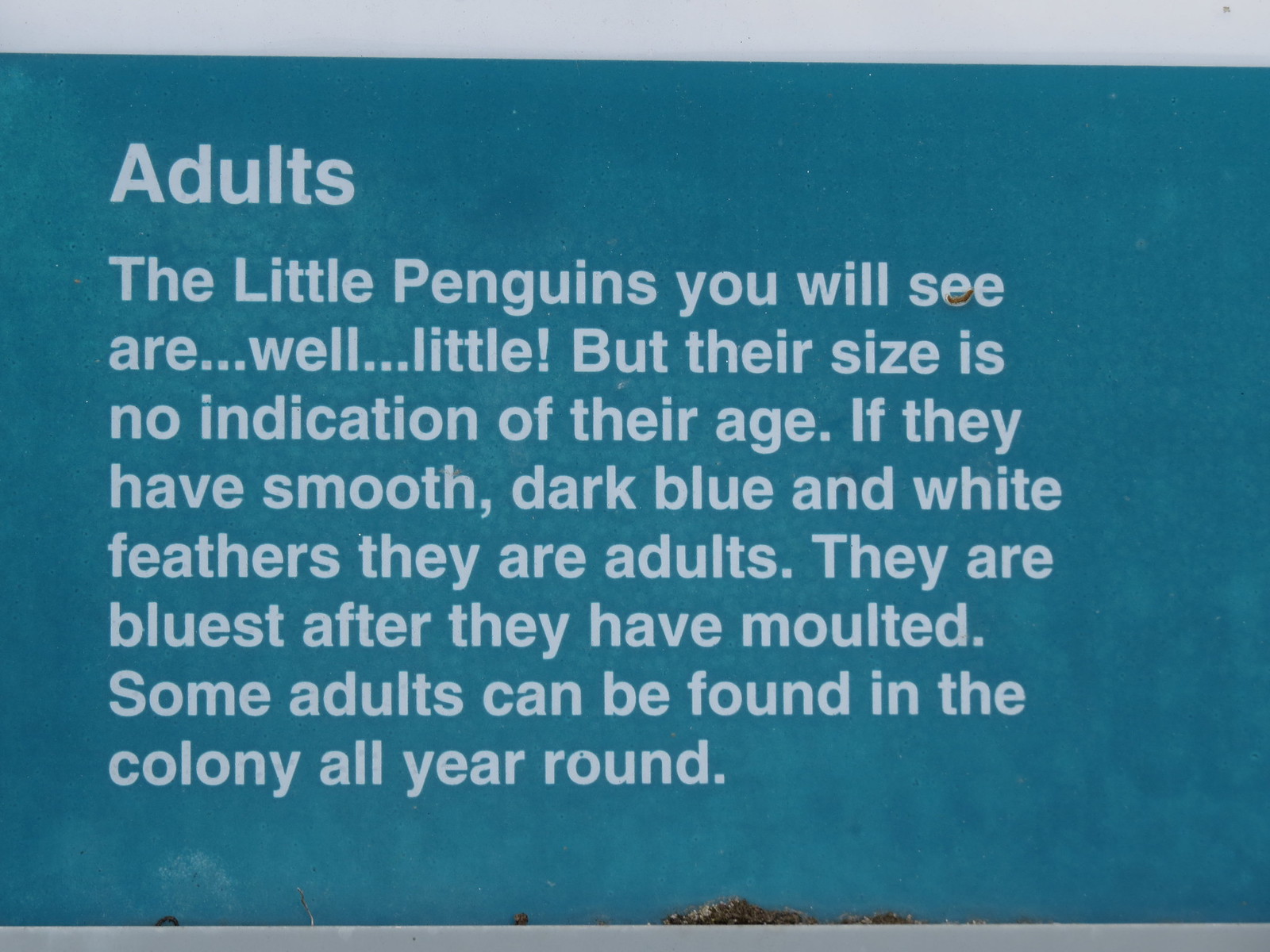The display, likely a placard at a zoo or an aquarium, features a predominantly turquoise or deep sea blue background with a paragraph written in white text under the bold title "ADULTS." This text describes the characteristics of adult penguins, emphasizing that their small size does not indicate their age. Notably, adult penguins are identified by their smooth, dark blue and white feathers, which appear their bluest after molting. Additionally, the placard informs visitors that adult penguins can be seen in the colony throughout the year. The overall design includes a gray band along the top and bottom, and the text has a slight bluish or turquoise tint, adding to the visual appeal.